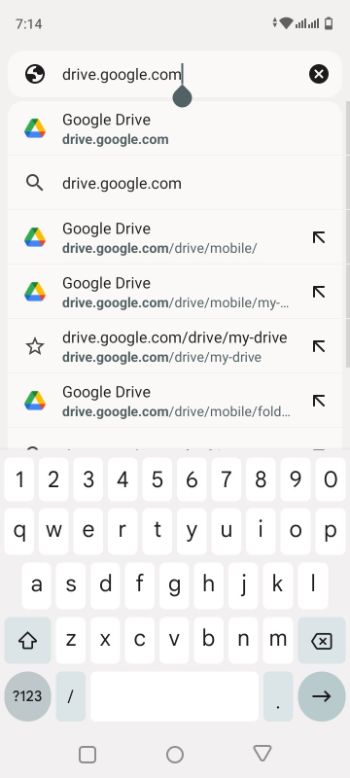The image depicts a cell phone screen displaying a webpage with Wi-Fi enabled while the battery is low. The URL shown is "drive.google.com," with a cursor immediately following the "m" in ".com." An "X" icon appears next to the URL, allowing users to close the page. Below this, the page features multiple instances of "Google Drive" and various URLs associated with it, including "drive.google.com," "drive.google.com/drive/mobile," and "drive.google.com/drive/my-drive." 

The screen also shows part of the URL "drive.google.com/drive/my-drive," and an incomplete URL "drive.google.com/drive/mobile/full..." suggesting longer links. At the bottom of the screen is a white keyboard with black font, featuring gray keys for functions such as backspace, numbers, a right arrow, forward slash, and period. The cell phone navigation icons are situated at the very bottom of the screen.